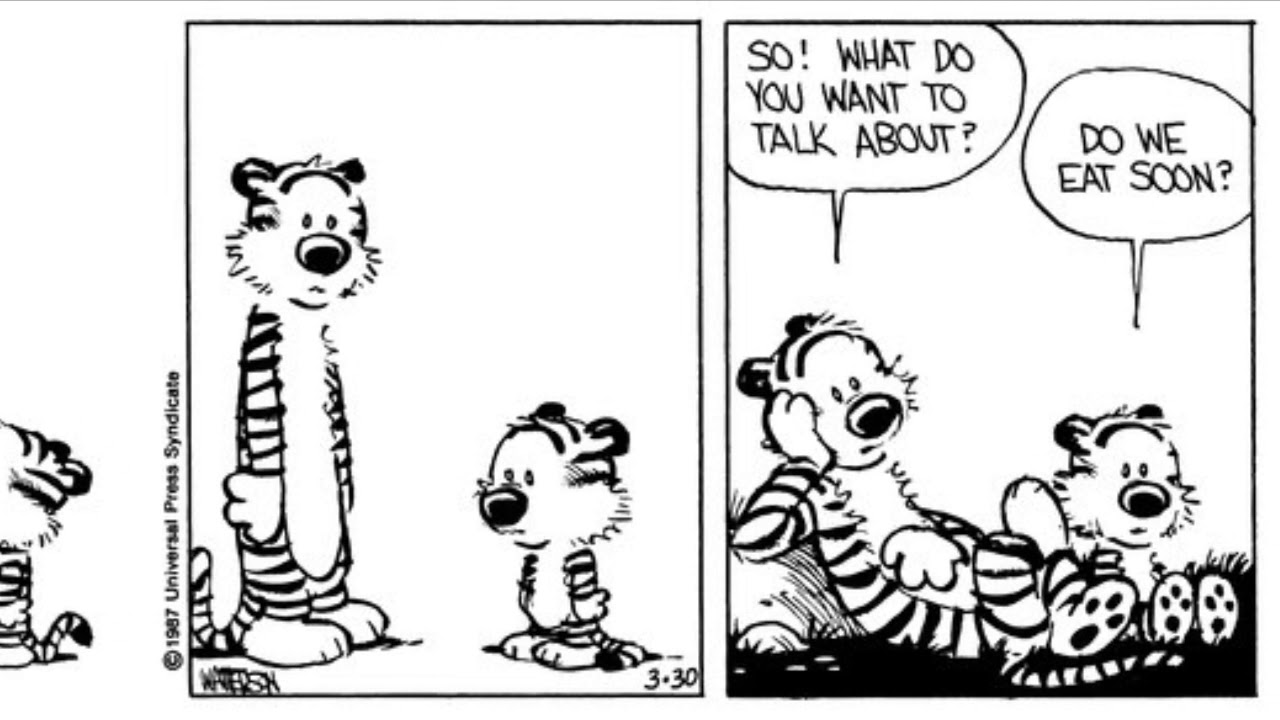This comic strip, titled "1987 Universal Press Syndicate" and created by Bill Watterson, features two tigers—a tall adult tiger and a smaller baby tiger—in a black and white format. The first panel presents both tigers standing side by side. The adult tiger, with distinct striped patterns and a white face, black nose, white stomach, hands, and feet, looks attentively at the baby tiger who appears to be gazing down. The number "3-30" is visible in this frame.

In the second panel, the adult tiger, still maintaining his characteristic features, places an arm on his head and appears to be leaning against a rock while they both sit on black grass with a white background. The larger tiger asks, "So what do you want to talk about?", while the smaller tiger, mirroring the adult's coloring and button nose, responds with, "Do we eat soon?" This scene captures a moment of interaction and curiosity between the two, embodying a relaxed and ponderous atmosphere.